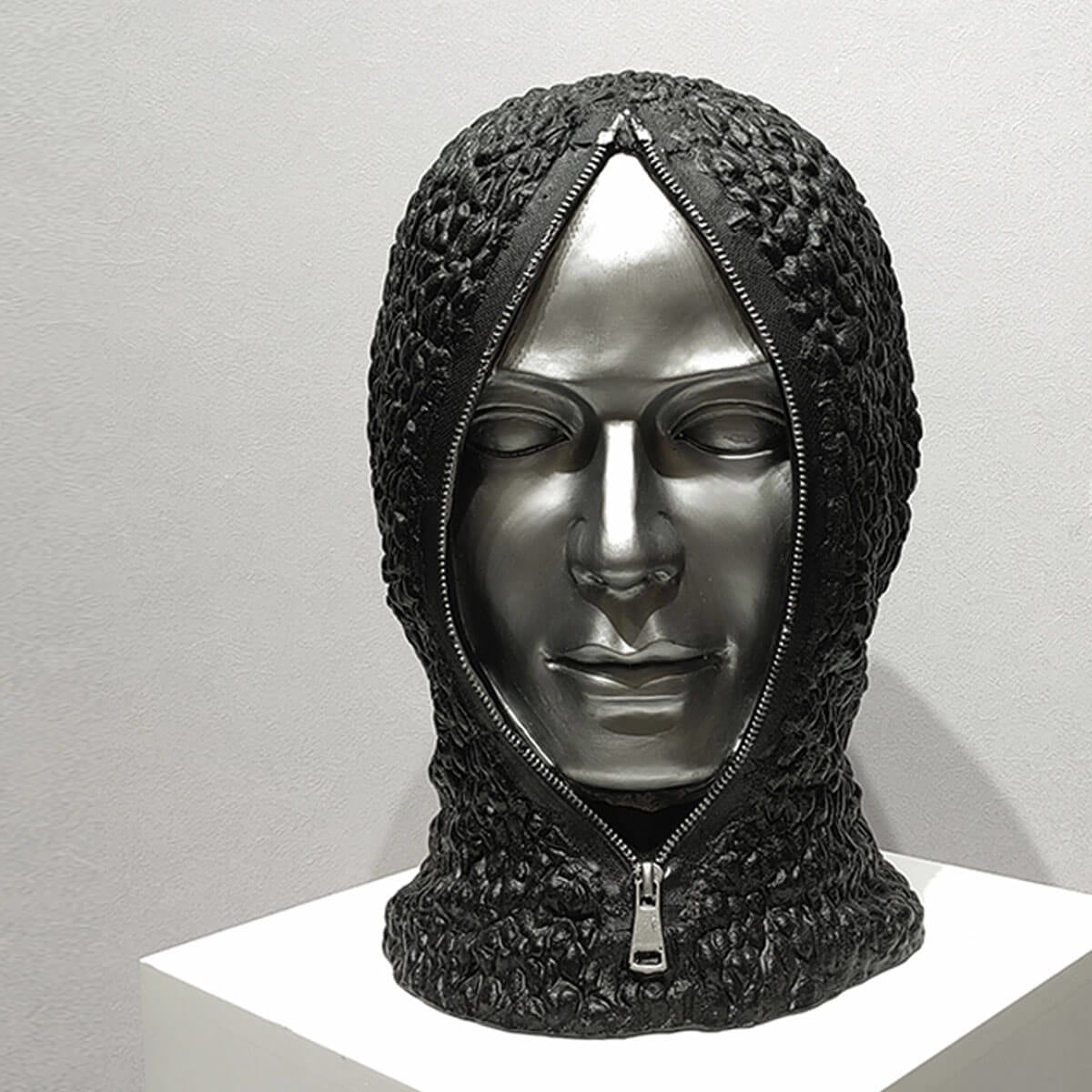The image depicts a bust of a human head, artfully displayed on a white pedestal with a light gray background. The metallic head, crafted from what appears to be stainless steel, features closed eyes and a serene expression. Draped over the head is a black textured hood that closely resembles a ski mask or an S&M face mask, complete with a zipper that runs from the top of the forehead down below the chin. This zipper is currently open, revealing the smooth, silver surface of the face beneath. The scene is meticulously arranged and suggests a museum exhibit or a high-end product presentation, emphasizing the artistic and perhaps provocative nature of the piece.